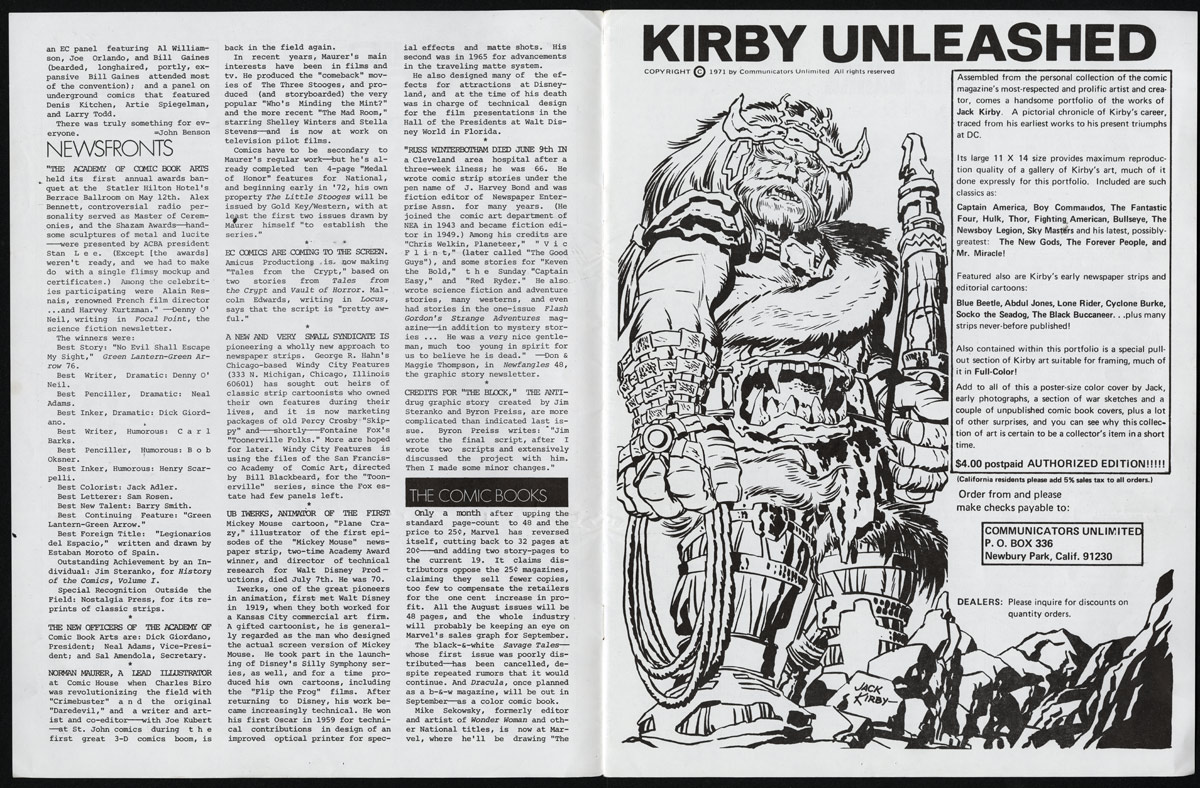The image features an open magazine displaying a two-page spread primarily in black and white. The left page contains three long columns of text, interspersed with two distinct headings: "News Fronts" at the top left and "The Comic Books" towards the bottom of the third column. The right page showcases a bold heading at the top in black letters, "Kirby Unleashed." Beneath the title is a detailed black-and-white drawing of a stocky, angry-looking troll or Viking figure with abundant hair. The figure's distinctive feature includes an open mouth with fangs located where his belly should be. In his hands, he wields a rope on the left and a club or stick on the right. Positioned around him are some rendered rocks and mountains. The page also contains columns of text, one situated to the right of the illustration, providing additional context or articles related to "Kirby Unleashed".